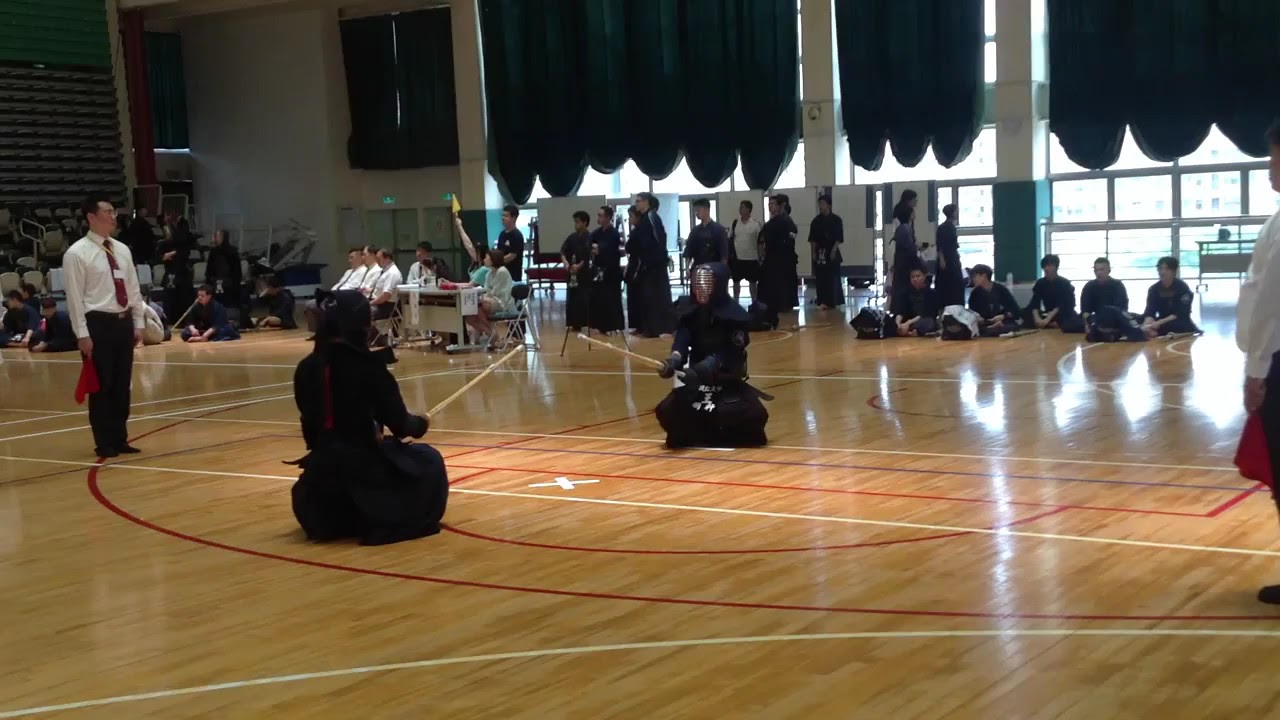The image captures a detailed scene of a martial arts competition taking place inside a gymnasium with a shiny, patterned wooden floor that bears the markings of a basketball court. At the center of the image, two competitors are in a squatting position facing each other, equipped with bamboo swords. They are dressed in full black protective armor, including large shoulder pads and metal face shields. Around them, the scene is bustling with activity; along the wall, numerous spectators, mostly martial artists in black uniforms, are either sitting or standing. Additionally, on the sides of the central area, two referees are standing, identifiable by their white shirts, black trousers, and red ties, each holding a red handkerchief. Further in the background, there's a person seated at a table with a yellow flag, alongside large white pillars and windows, adding to the ambiance of the gymnasium. The referees and spectators keenly observe the participants, capturing the intensity and anticipation of the moment as the competitors prepare to engage.